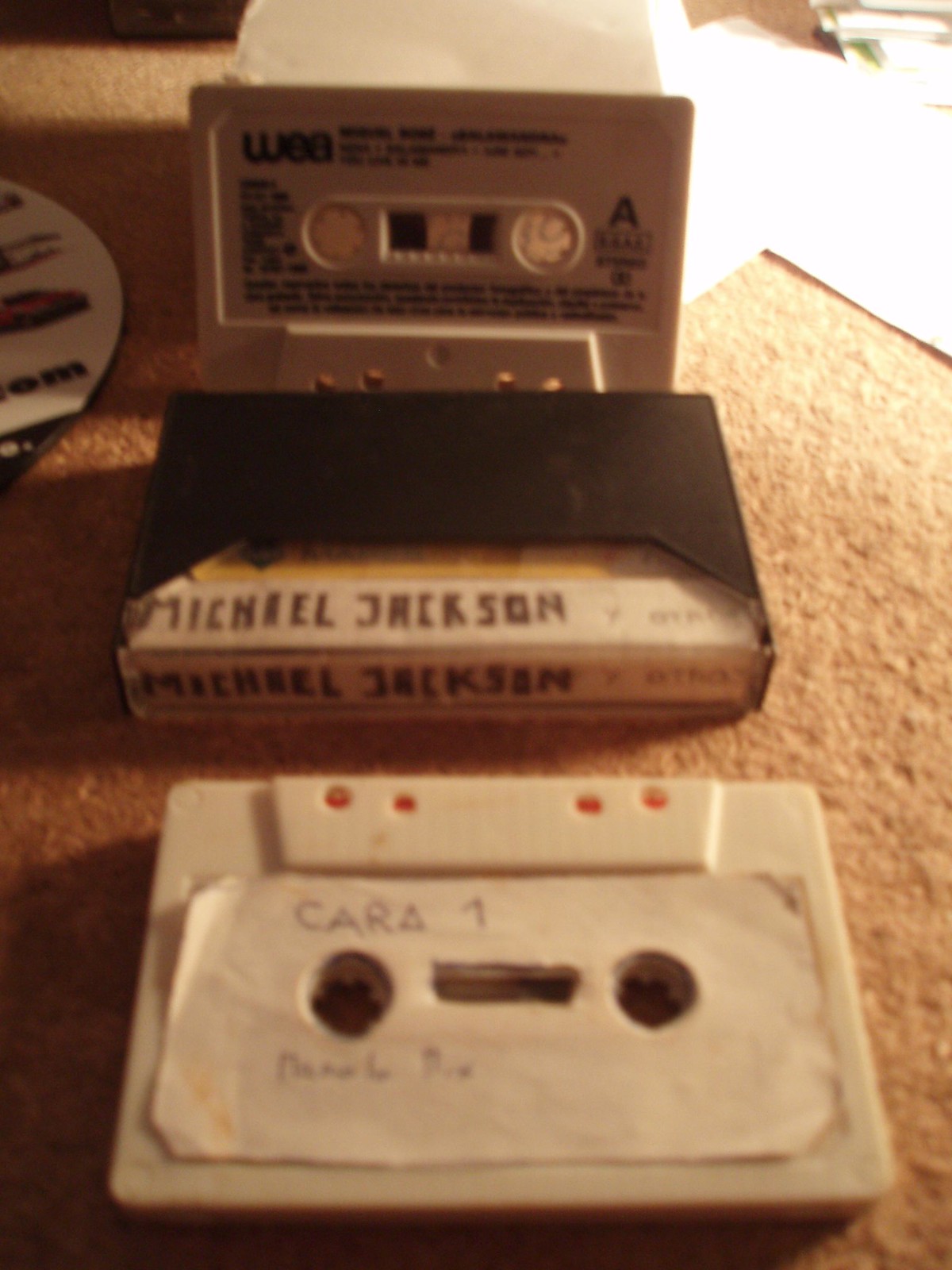The photograph depicts three cassettes arranged vertically on a light brown carpet. The top cassette is white, standing upright, and features a large letter 'A' on its lower right corner; it appears to have "WEA" written on the top left. Below it, there is a black cassette case flipped upside down, with "Michael Jackson" written in two places, suggesting it originally housed a Michael Jackson tape. At the bottom of the arrangement is another white cassette without a case, displaying a paper label that reads "Cara 1." In the upper left and right corners of the image, there are pieces of illegible paper and possibly the edge of a CD. These cassettes, popular in the 70s and 80s, evoke nostalgia for a time when they were commonly used, despite occasionally getting tangled in tape players.